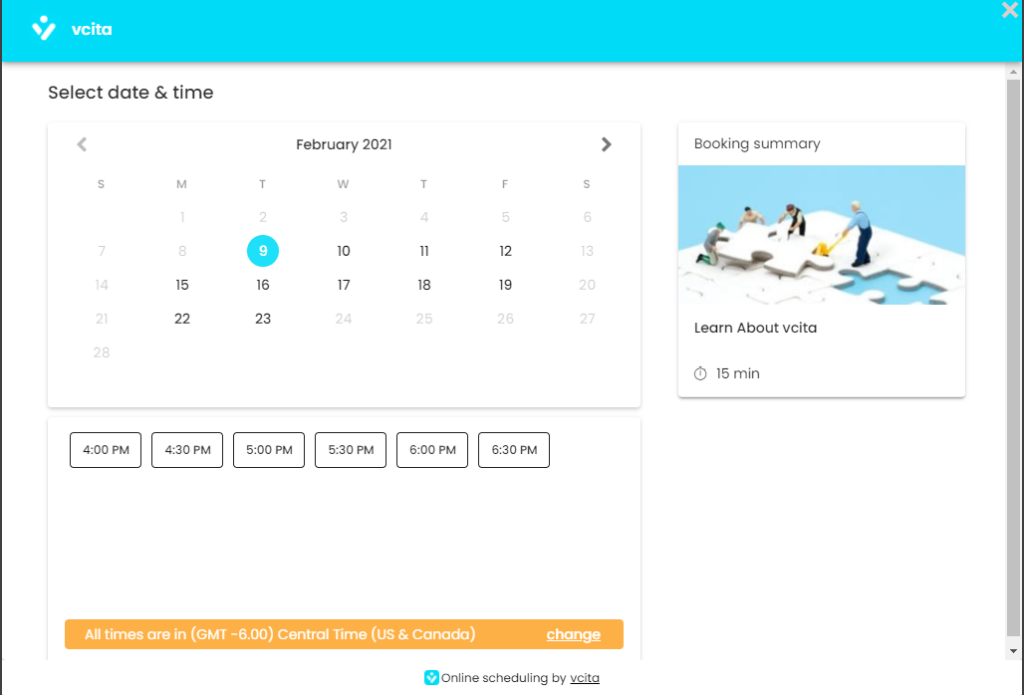The screenshot is from a scheduling website called VCITA. At the top of the page, the heading "Select Date and Time" is prominently displayed, guiding users through the booking process. Directly below, a calendar for the month of February 2021 is shown with various dates, some of which are grayed out and not selectable. Specifically, all Saturdays and Sundays, along with the days leading up to February 9th, are unavailable.

Dates that are selectable, bolded in dark black font, include February 9th, 10th, 11th, 12th, 15th, 16th, 17th, 18th, 19th, 22nd, and the 23rd. The date currently selected is February 9th, marked by a blue circle around it. Below the calendar, there are available time slots listed for the selected date: 4:00 PM, 4:30 PM, 5:00 PM, 5:30 PM, 6:00 PM, and 6:30 PM. An orange notification beneath these slots indicates, "All times are in GMT-6 Central Time (US & Canada)," with an option to change the timezone.

In smaller font at the bottom of the scheduler, it states, "Online scheduling by VCITA." On the right side of the screen, within the "Booking Summary" section, there is an image of people holding puzzle pieces along with the caption "Learn by VCITA." The booking summary specifies the duration of the meeting as "15 minutes."